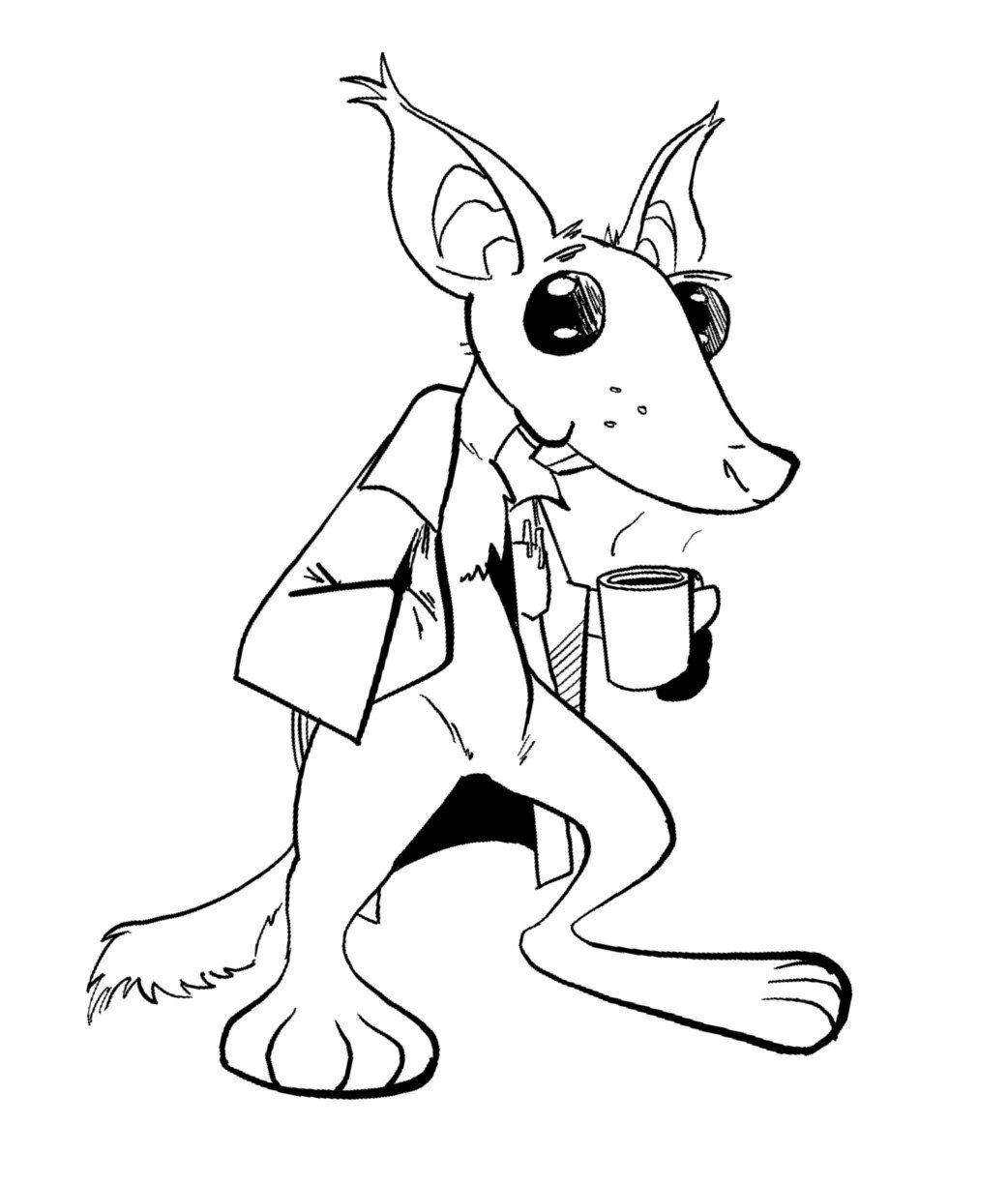This detailed black-and-white line drawing features a humanoid rodent-like creature standing upright on two legs. The creature wears a long lab coat adorned with pins in the pocket, suggesting a role akin to a doctor or lab technician. It holds a coffee mug with steam rising from it in its left hand, which appears on the right side of the image. The rodent has distinct characteristics: bulging black eyes, a long snout, and large ears with tufts at the ends. Its prominent front teeth jut out from under its jaw, and it has a bushy, possibly spiky, tail. The legs resemble those of a kangaroo with elongated feet sporting four toes. The eyes appear watery, giving it a somewhat thoughtful or weary expression. Overall, the image depicts an anthropomorphic rodent engaging in human-like behavior, set in a simplistic, monochromatic design.